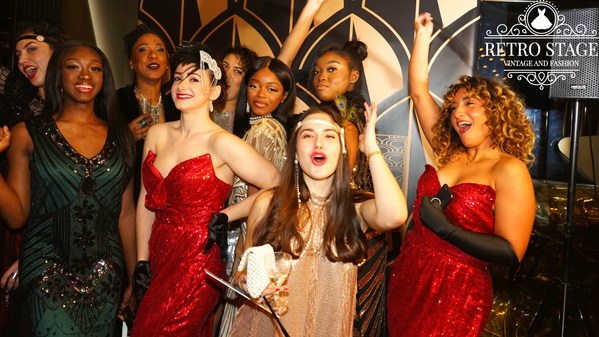In this vibrant and joyous image, nine women, possibly models, stand posing at a glitzy fashion event. They exude happiness, smiling and cheering, and are dressed in an array of elegant, vintage-style costumes that evoke a period fashion. The women, representing a diverse range of skin tones, include those with dark brown and white skin, and possibly mixed race.

To the right, a prominent sign on a black tripod reads “Retro Stage Vintage and Fashion” in white lettering, suggesting the setting may be a fashion show. Two women grace the scene in striking red ball gowns, while another on the left wears a stunning green and black dress. The central figure gleams in a light golden dress, holding a glass of wine in her right hand and raising her left hand in celebration. Nearby, another woman in a gold-colored dress joins the festive mood.

The attire varies from dresses with high collars to those with no collars, some adorned with headbands and lacy accessories, reminiscent of high fashion from America's early 60s. Their shared excitement and elegant attire paint a vivid picture of a jubilant moment at a glamorous event.